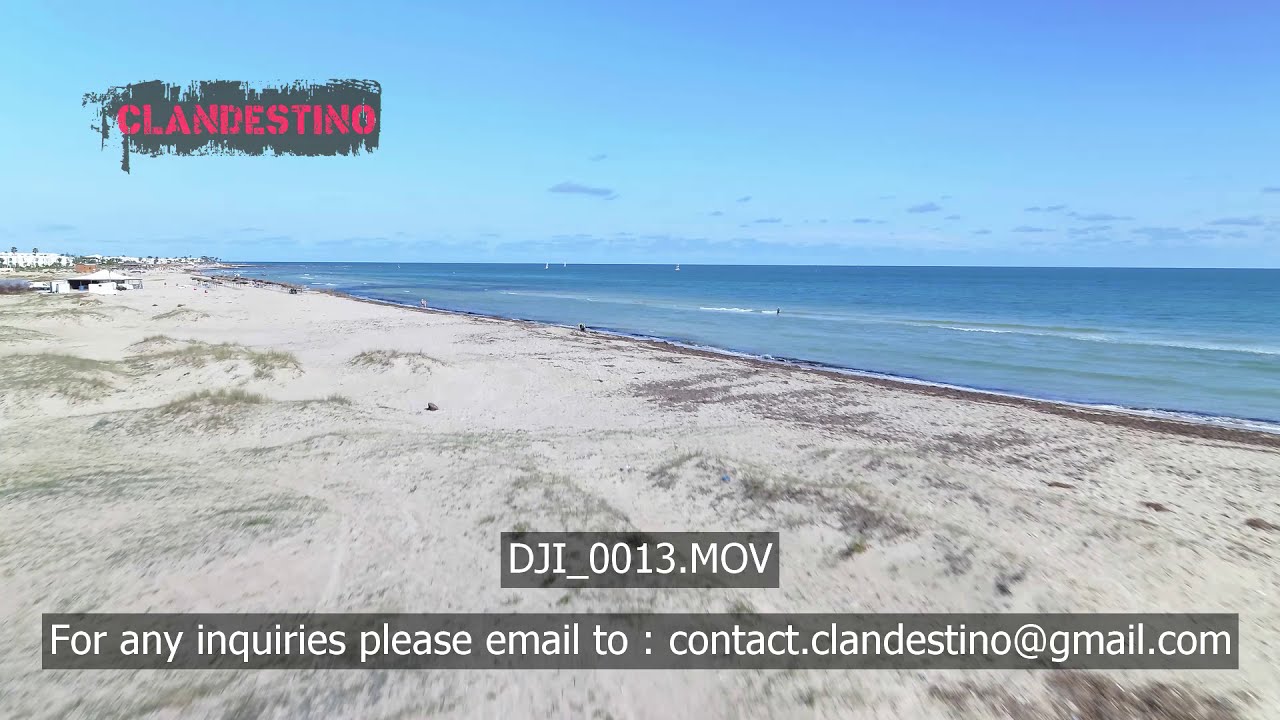This image appears to be a screenshot from a video, capturing a serene beach scene. The vantage point places us on the sandy shoreline, with the ocean to the right, showcasing its gradient from a pale blue near the shore to a deeper blue as it extends outward. Low-lying waves gently lap at the beach, where sparse vegetation, including small sand mounds and patches of green grass, are visible. The day is clear with a bright blue sky and a few thin clouds on the horizon. Scattered beachgoers and small white structures dot the scene, leading up to a line of hotels in the distance. The upper left corner of the image features a spray-painted-style logo reading "Clandestino" in red text. The bottom part of the image contains the video file designation "DJI_0013.MOV" and contact information, directing inquiries to "contact.clandestino@gmail.com."